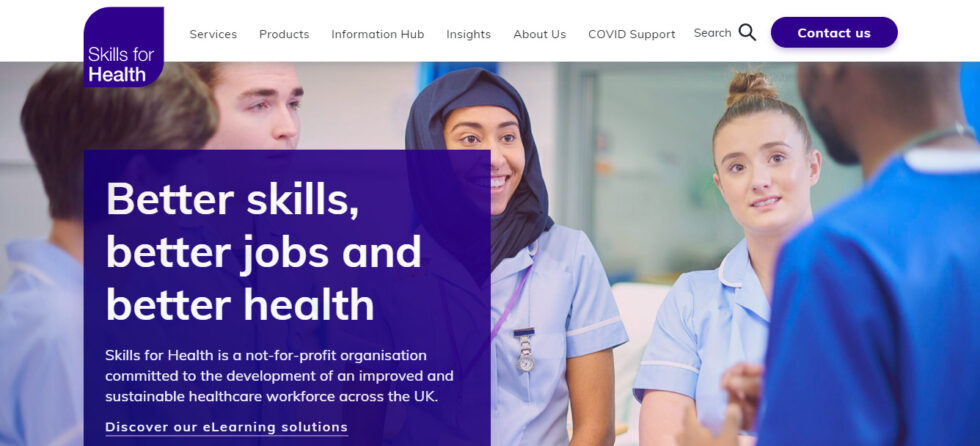A desktop screenshot showcasing the website for "Skills for Health." The website's header features a distinctive purple-colored logo on the top left, with the text "Skills for Health" inscribed within an irregularly shaped square that has a curved top left and bottom right corner, while the top right and bottom left corners are pointed. Adjacent to the logo is a navigation bar with several tabs labeled "Services," "Products," "Information Hub," "Insights," "About Us," "COVID Support," and a search icon resembling a magnifying glass. A prominent purple pill-shaped button on the right side of the navigation bar reads "Contact Us."

Below the header, the main content area displays a background image featuring several nurses. At the center is a female nurse wearing a traditional Muslim headdress flanked by two Caucasian nurses. One male nurse on the far left has light skin and faces away from the camera, while another male nurse on the far right, dressed in a blue uniform, appears to be African American.

On the middle left side of the screen, a compelling message states, "Better skills, better jobs, better health." Beneath this statement, the website describes "Skills for Health" as a not-for-profit organization dedicated to developing a skilled and sustainable healthcare workforce across the UK. A clickable hyperlink below invites viewers to "Discover our e-learning solutions."